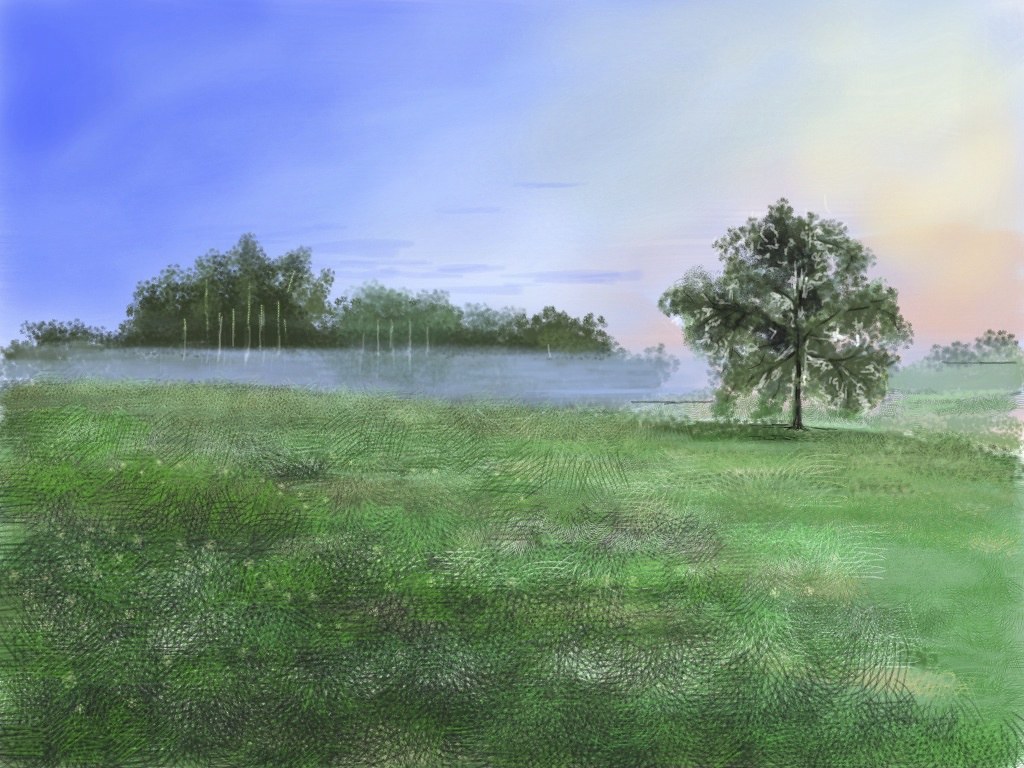This artwork is a stunning landscape painting or digital illustration, predominantly composed of various shades of green that cover approximately 60% of the image. The scene depicts a serene hillside, dominated on the right side by a solitary tree. This tree is characterized by its long, graceful branches that almost sweep the ground, adorned with lush foliage and supported by a slender brown trunk.

In the background, behind the tree, there's a captivating fog or a wispy blue effect that veils a further landscape of trees, lending a mysterious and ethereal quality to the scene. This misty element effectively obscures the distant trees, adding depth and intrigue to the composition.

The upper section of the image, occupying around 30% of the space, is devoted to a sky that transitions elegantly between blue and pink hues, suggestive of a sunset. The sky is also punctuated by delicate white clouds, enhancing the peaceful atmosphere. Toward the right side, the sun appears to be setting, casting a gentle glow across the sky, while the remainder of the sky remains relatively undisturbed with wispy clouds.

The hillside itself is a tapestry of assorted greens, ranging from light to dark, interspersed with touches of brown and light yellow, which add texture and richness to the landscape. The harmonious blend of colors and elements creates a vividly detailed and immersive image.